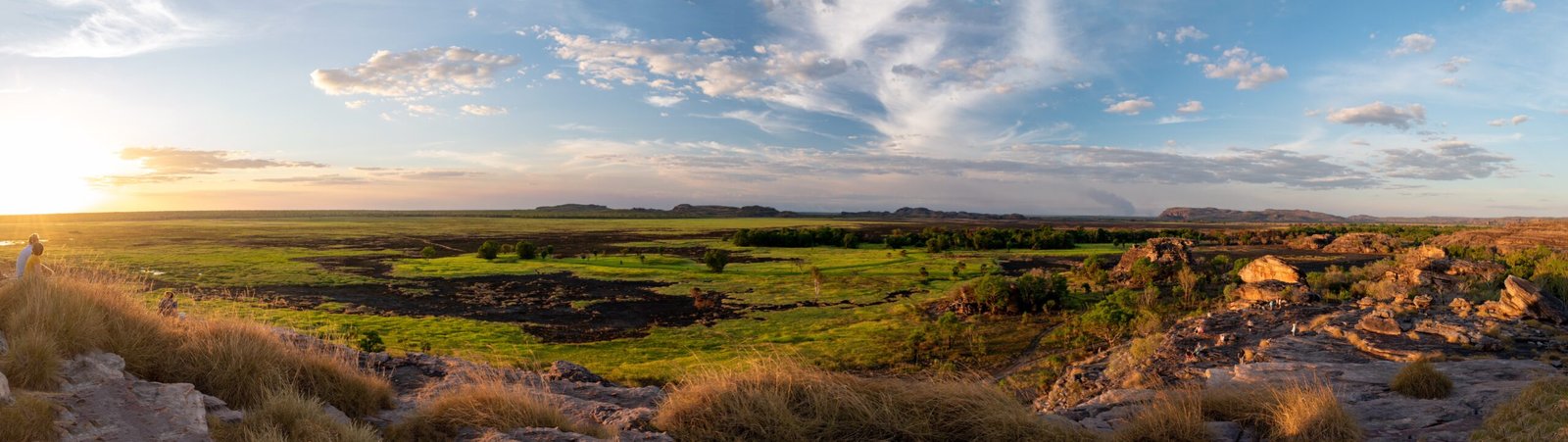In this panoramic image of a rural outdoor scene, a clear blue sky is scattered with clouds, featuring wispy formations near the top and more consolidated cloud cover stretching across the middle. The left side of the image reveals a sun low on the horizon, casting light across a field that's lush with green grass, turning rocky and dry towards the right. The field is predominantly grassy and dotted with weeds resembling hay, particularly in the foreground. To the right, the terrain becomes rockier with patches of dirt.

Two individuals in blue and yellow shirts stand or sit atop a grassy area on the left side, facing right, with sunlight illuminating their location. A closer inspection reveals more people dispersed throughout, including some who are faintly visible walking around the rocky flat area on the right. In the distance, towering rock formations stand elevated above the plains, further accentuating the rugged beauty of the landscape. The sky transitions from light to darker hues across the frame, capturing the depth and expansive nature of the scene through what appears to be a high-resolution, possibly VR-captured image.